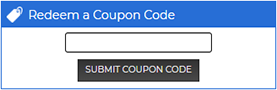A screenshot of an online shopping platform's coupon redemption section. The image features a blank, empty text field where users can enter their coupon code. Below the text field is a "Submit Coupon Code" button with a gray background. The entire coupon redemption section is framed by a blue square, emphasizing the area where users need to focus to apply their coupon.